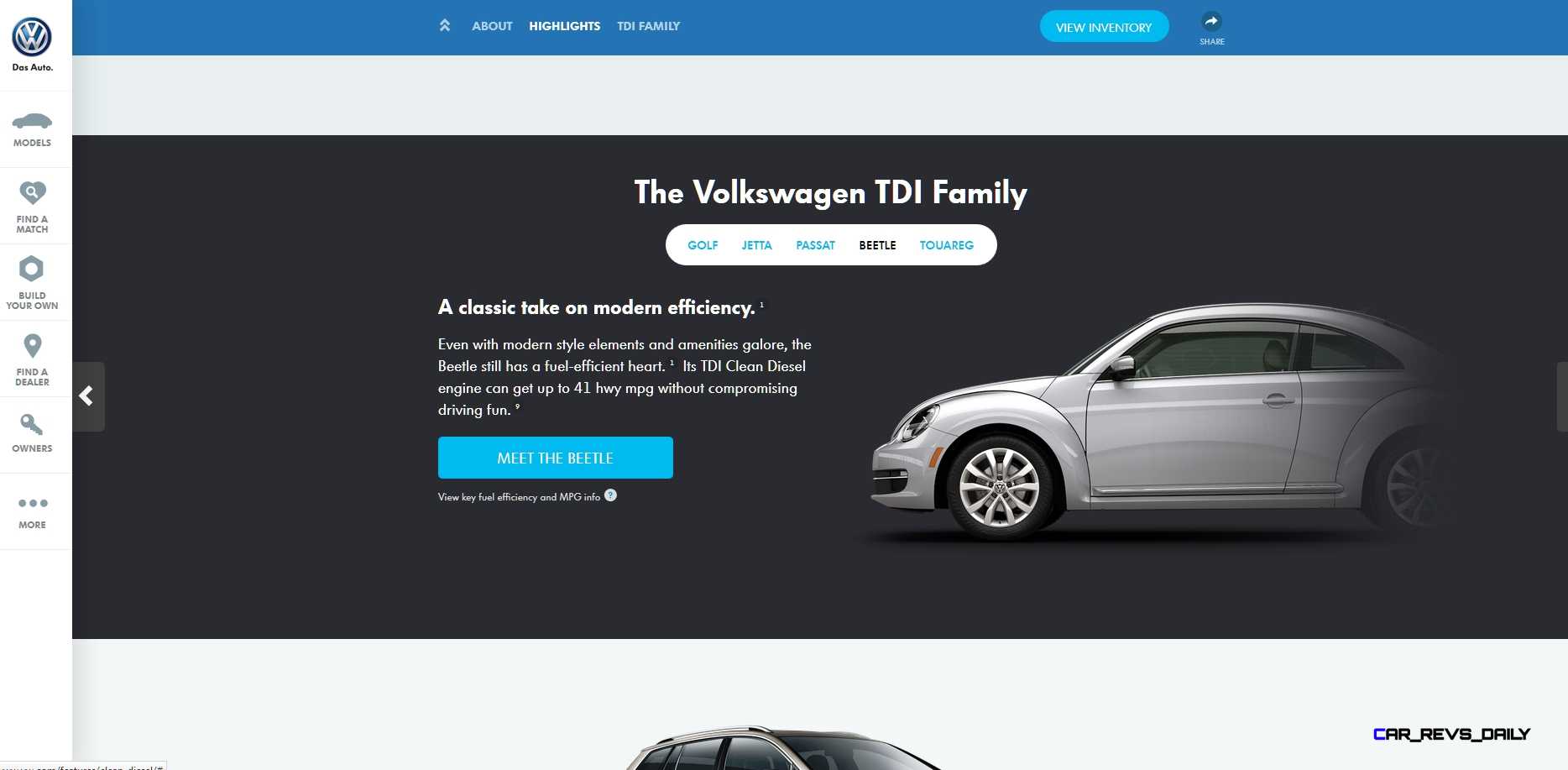This is a website for the Volkswagen car company. In the top left corner, the Volkswagen badge logo is prominently displayed. The logo features an interlocking "V" and "W" within a circle, rendered with a silver inner color and a blue outline. Below the badge, the words "Das Auto" are inscribed. The website’s top navigation bar is blue and contains three tabs: "Highlights," "TDI Family," and "View Inventory," with the latter positioned on the right side.

Central to the main page is an image of a silver Volkswagen Beetle. Above the car, the text reads "Volkswagen TDI Family," and beneath this heading, there's a white pill-shaped menu bar listing the model names: Golf, Jetta, Passat, Beetle, and Touareg. The "Beetle" is distinctively written in black, different from the others.

Accompanying the image, white text describes the Beetle as "A classic take on modern efficiency." Below this description, there are four additional lines of white text and a blue call-to-action button.